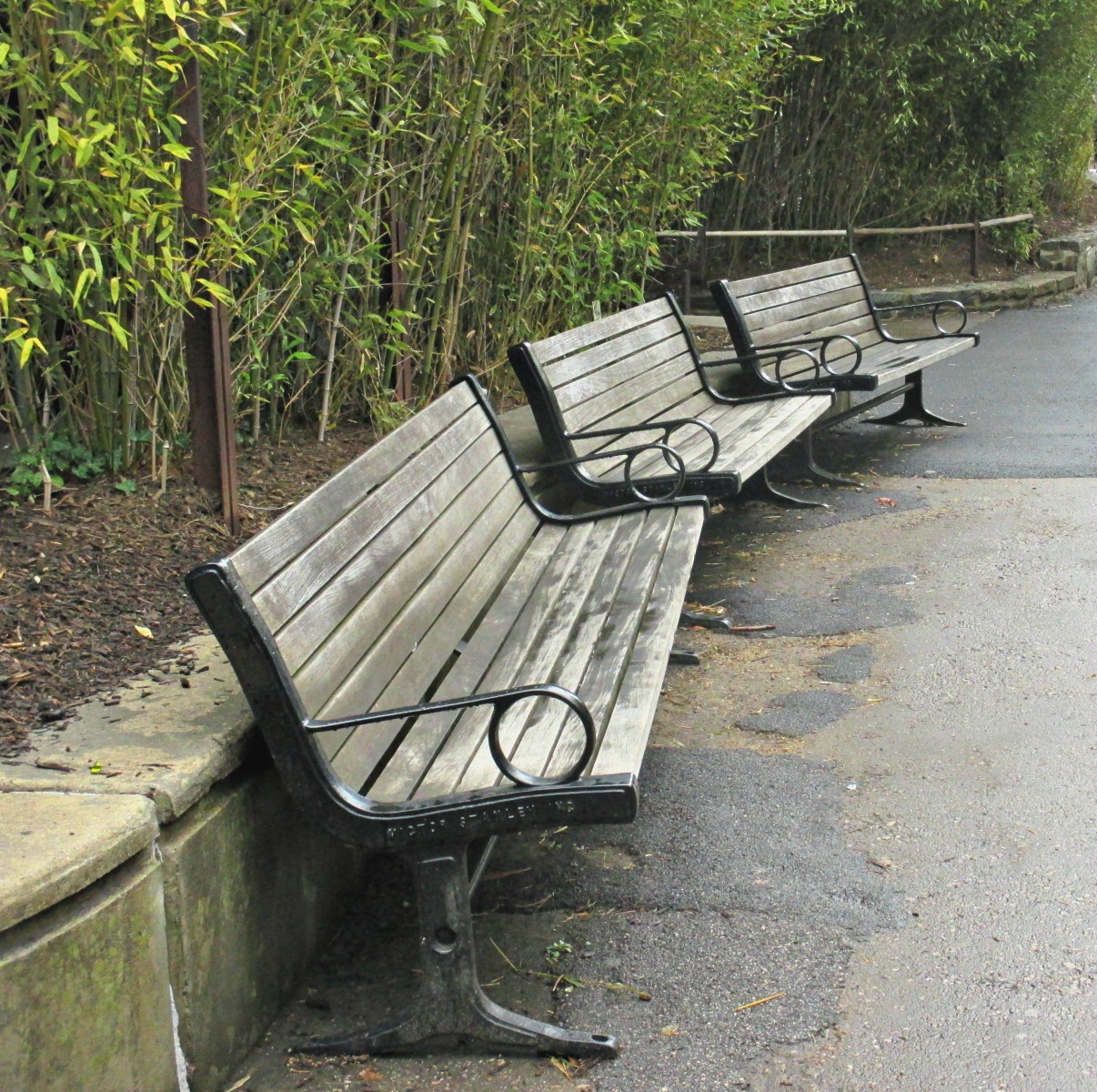This outdoor daytime photograph captures a serene park walkway under an overcast sky, dotted with greenery. The focal point consists of three weathered wooden park benches with wrought iron frames, painted black and showing signs of age. These benches are aligned in a row, positioned diagonally, and backed against a four-foot-tall concrete retaining wall. Behind the wall, a dense thicket of bamboo and various plants provides a lush backdrop. The pathway—a wide sidewalk of macadam—intersects with another path beyond the third bench, indicating a well-trafficked park or a sanctuary-like area. The benches' worn grayish-brown slats hint at years of outdoor exposure, while the muted light casts a calm, serene ambiance across the scene, devoid of shadows or sun.